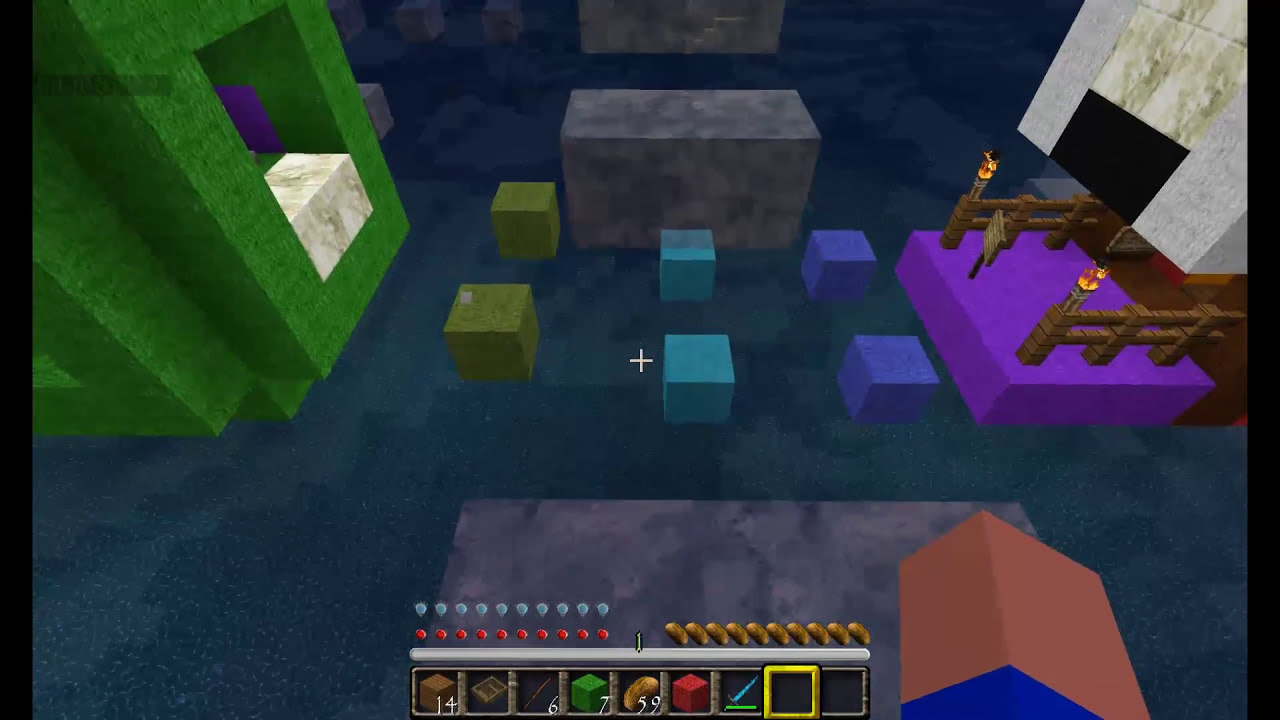This is a screenshot from a primitive video game, possibly a construction template or a Minecraft-like environment. The scene appears to be set inside a stone castle or similar structure. The floor is a blue and gray tiled pattern, scattered with numerous geometric shapes including green, blue, and purple cubes, as well as gray prisms that resemble altars or cabinets. On the left side, there's a green structure featuring stacked cubes and a white cube on top. In the middle of the room, there are smaller yellow, blue, and violet blocks that look like stools or chairs leading up to a purple altar with wooden sides and computer-generated flames. The scene is further accented by fencing with torches and other geometric blocks at the bottom. 

An inventory control panel is displayed at the bottom of the screen, showing various collected items and their quantities: 14 brown boxes, 6 books, 7 green blocks, and 59 copper coins. Additional design elements include a small gray, unreadable watermark, a white crosshair in the center, and various avatar-like icons, possibly representing scores or item counts. The top right of the screen also shows some icons resembling potatoes along with a series of blue and red dots. Overall, the image depicts a rudimentary but imaginative virtual space with elements indicative of classic block-styled video games.